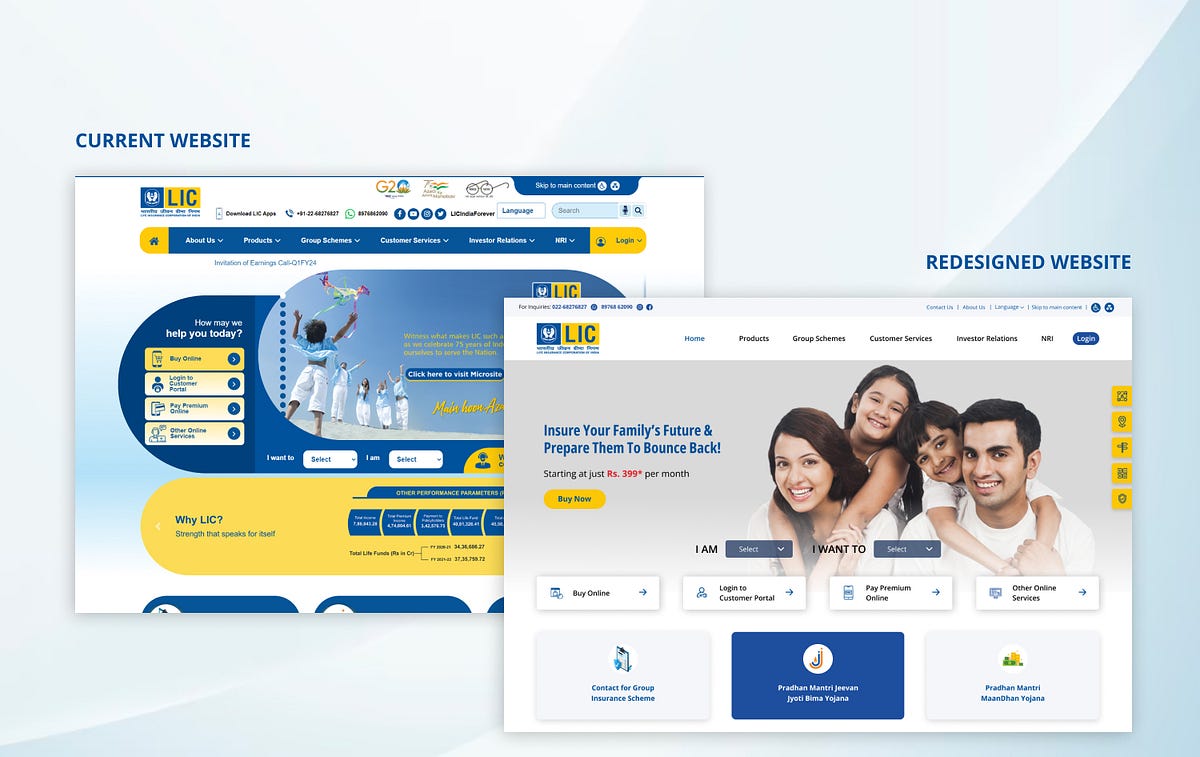### Caption for the Image: 

This image compares two versions of a website from the same company. The left side showcases the **Current Website** with a predominantly yellow-orange background and blue text. At the top, it features the blue text "LIC" followed by options such as "Download LIC Apps," a phone number, and a search text box labeled "Language." Below this, there are several navigation buttons, including "Home," "About Us," "Products," "Group Schemes," "Customer Service," "Investor Relations," and a "Login" link. Under the navigation bar, a subtitle reads, "How may we help you today?" with options to "Buy Online," "Login to Customer Portal," "Pay Premium Online," and access other online services. The central image on this website shows a woman dressed in white capris and a short-sleeved blue shirt, taken from the back, with four others similarly dressed. A slogan towards the bottom states, "Why LIC? Strength That Speaks For Itself."

On the right side, the **Redesigned Website** features the slogan, "Ensure your family's future and prepare to bounce back." It includes an image of a younger man and woman, likely in their late twenties, both dressed in white. The woman is embracing a young girl from behind, and the man has a boy with his arms around his neck, creating a family-centric and modern appeal.